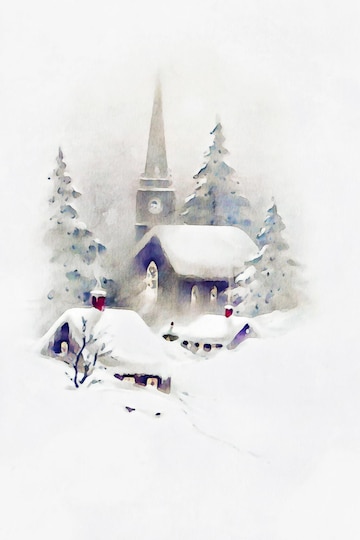This image is an 8x10 watercolor painting, resembling the delicate front of a Christmas card. Dominated by the soft white hues of heavy snowfall, the scene presents a serene rural village almost engulfed by winter's blanket. Central to the image is a tall church with a prominent steeple and bell tower, its dark, almost purple-black exterior standing out against the immaculate snow. The church features a large stained glass window above its front door, adding a touch of color to the monochromatic setting. Surrounding the church are three snow-laden fir trees of varying heights, adding depth and framing the focal point.

Scattered around the church are several structures, including smaller cottages and cabins nearly obscured by the snow, with roofs laden under what appears to be up to three feet of snow. One notable cottage has a distinctive red chimney poking out, capped with a dusting of snow. The scene is bathed in shades of white, blue, red, and gray, reflecting the calm and cold of a snowy day. All buildings are rendered almost inaccessible, buried so deeply that only the tops of windows and roofs peek out, highlighting the quiet isolation and beauty of this winter wonderland.